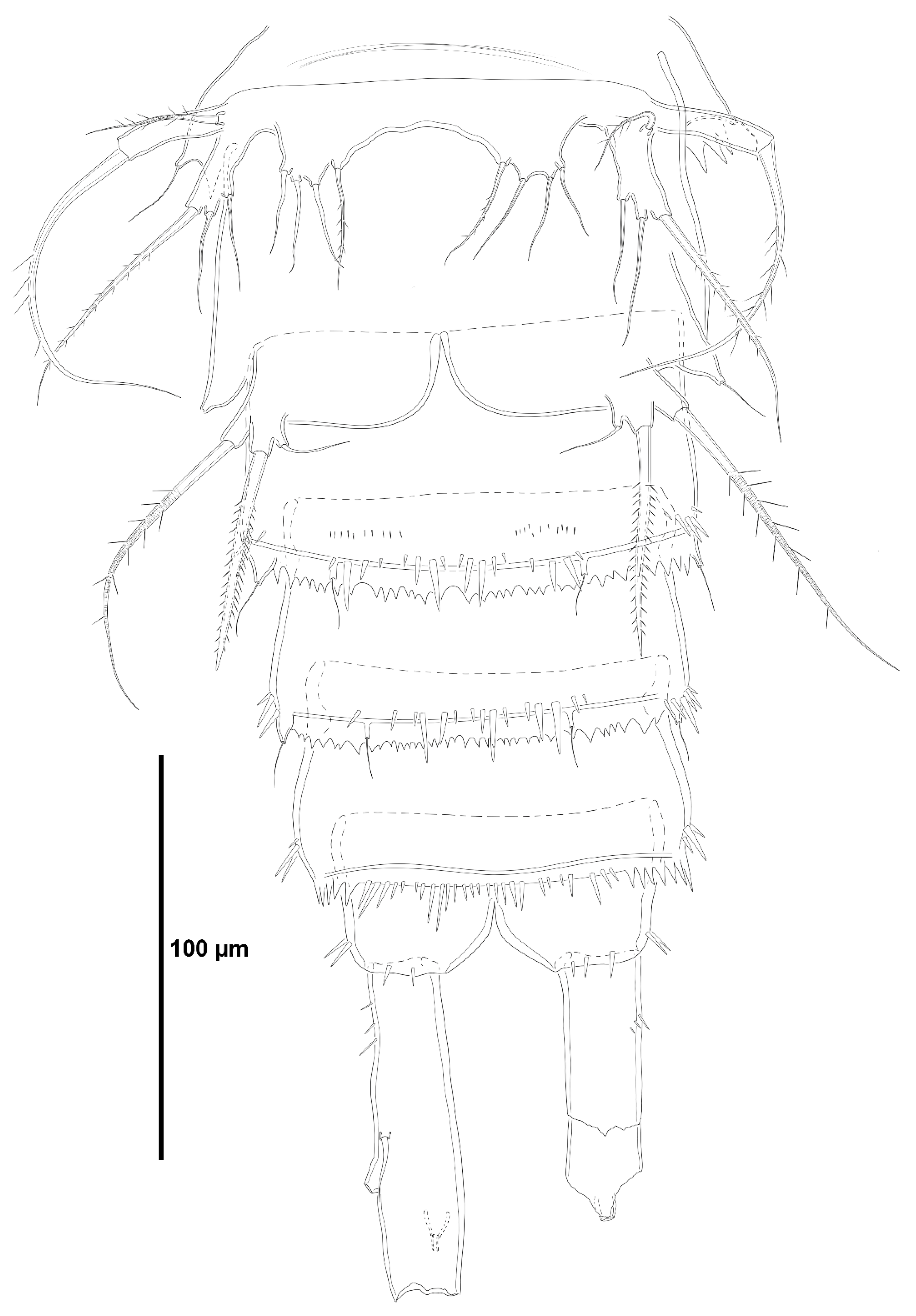This black and white illustration depicts an insect-like creature, reminiscent of a fly or bee. The image uses extremely fine and light lines, almost pencil-like in quality, to render the form against a stark white background. The creature features antennae adorned with hair-like spikes emerging from its head, two legs resembling hooves, and a layered torso. The drawing is somewhat abstract, with certain elements, such as the top of the head, appearing ambiguous, possibly suggesting glasses or another accessory. A notable element includes a horizontal black line on the left side of the image, accompanied by the number "100" and an upside-down "H" and "M," which appears to be a measuring scale extending near the bottom of the torso.